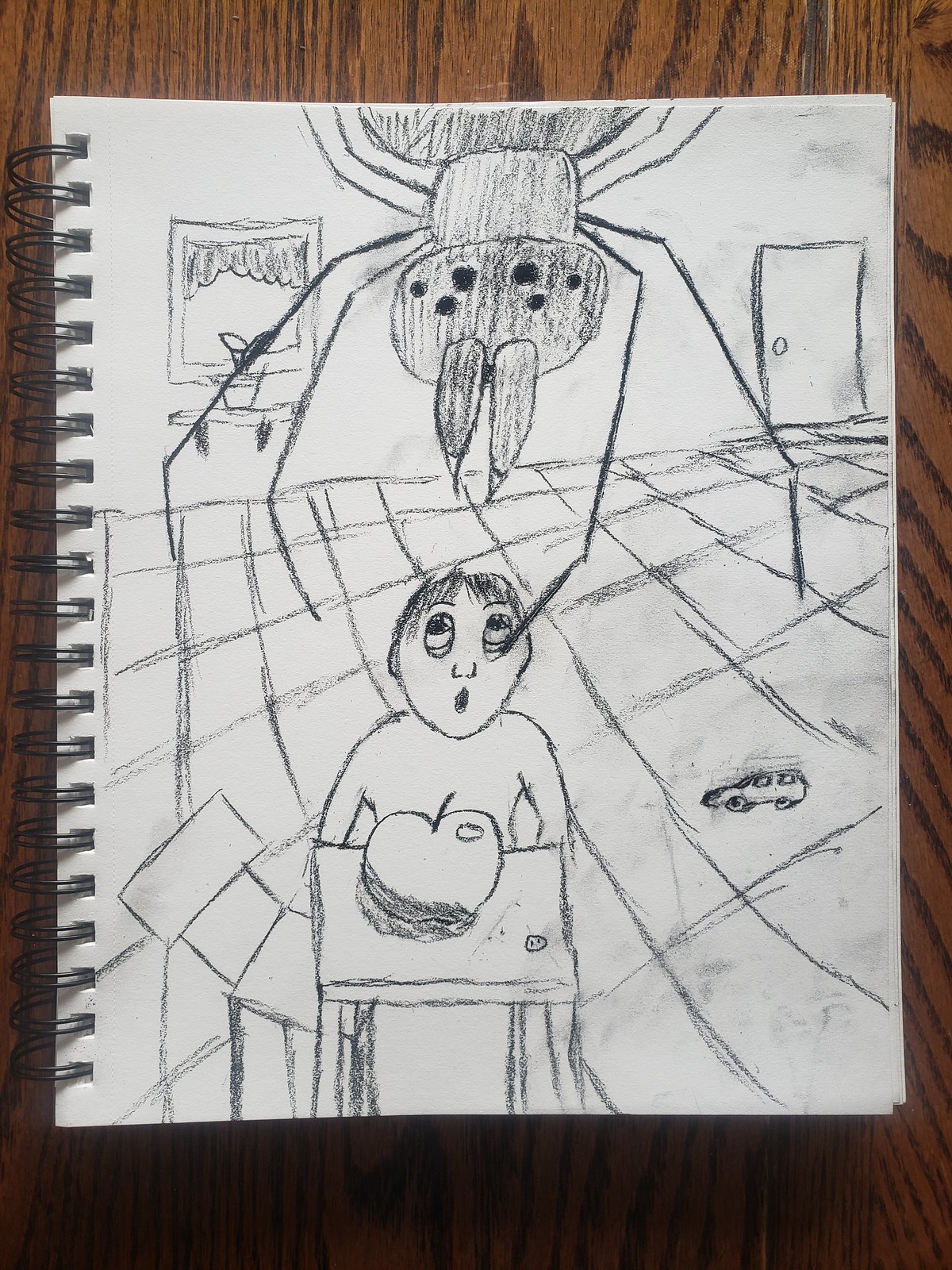The color photograph captures a detailed black and white pencil or charcoal drawing on white paper within a spiral-bound notebook, which rests on a medium to dark brown striped wooden tabletop. The sketch depicts a person with an open mouth, sitting at a desk and looking up at a massive spider descending from the ceiling. The spider, with menacingly long legs, six eyes, and giant fangs, has one of its legs extending down toward the person's eyelid. On the desk lies a large apple with a noticeable drop shadow. The background includes a window with curtains and a plant on the windowsill, a closed door to the left, and a checkered tile floor. A small toy car is drawn on the floor, adding extra detail to the scene.